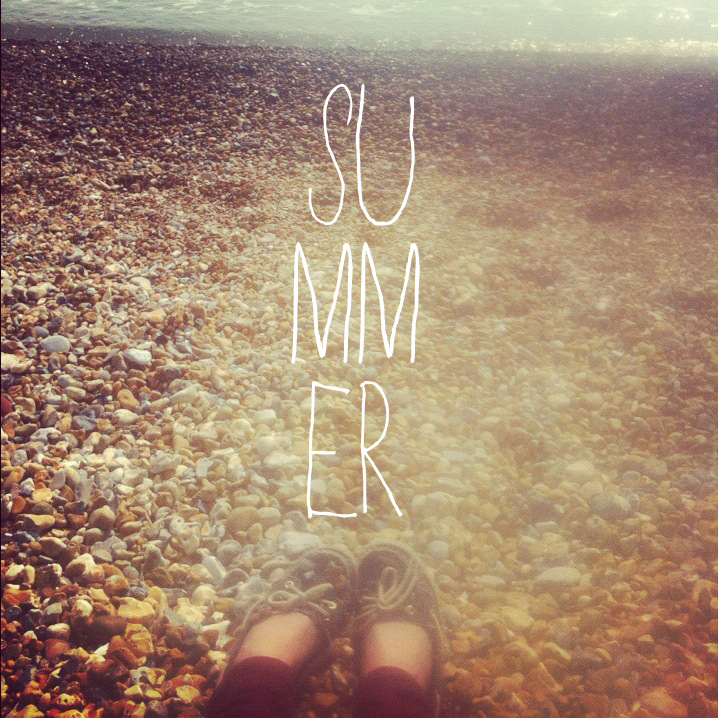The image is a stylized, slightly blurry photograph with a yellowish filter, capturing a serene seaside during daylight. It features a long shoreline covered in small, multicolored pebbles with hues of yellow, brown, red, and gray, all with soft, rounded edges. In the foreground, a pair of feet wearing blue moccasins with white laces are visible, and the hems of red pants are slightly seen above them. The water, a distant blue, gently laps against the pebble-laden shore. At the center of the image, the word "SUMMER" is written in thin white font, with the letters arranged vertically—S-U at the top, M-M in the middle, and E-R at the bottom.